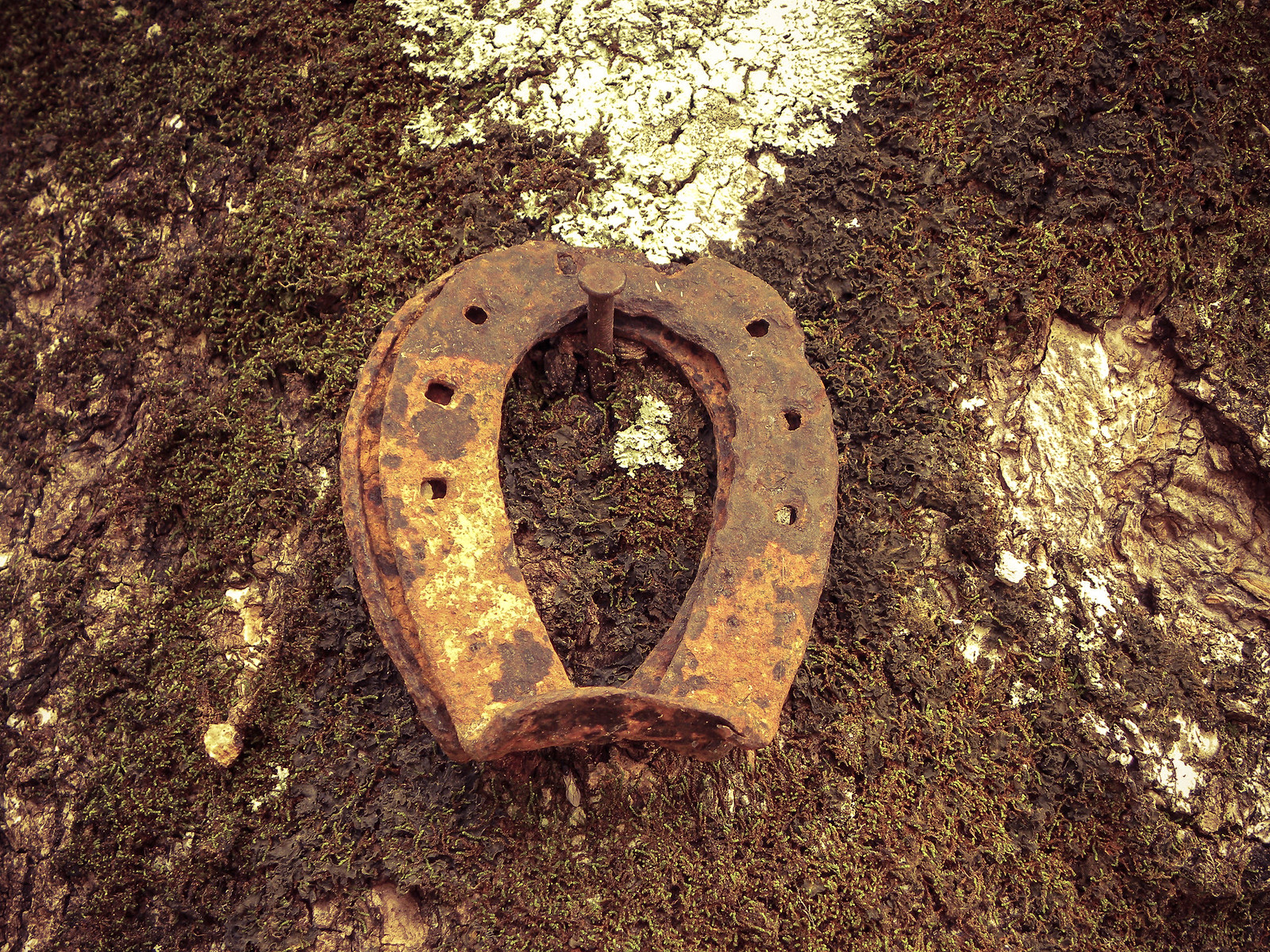The image presents an aerial view of a damp, dark brown ground with sparse green grass tufts. Centered is a rusted horseshoe attached to a large, equally rusted nail, appearing to be embedded in a tree trunk-like structure in the bottom right, complete with brown bark and potential moss. The horseshoe is unusually welded shut at its open ends, creating a flat lip that extends at a right angle. It features six evenly spaced holes along its arches, with an apparent chip at the top. Additionally, a distinct, light-reflecting area is visible at the top center of the frame, suggesting sunlight hitting the surface.